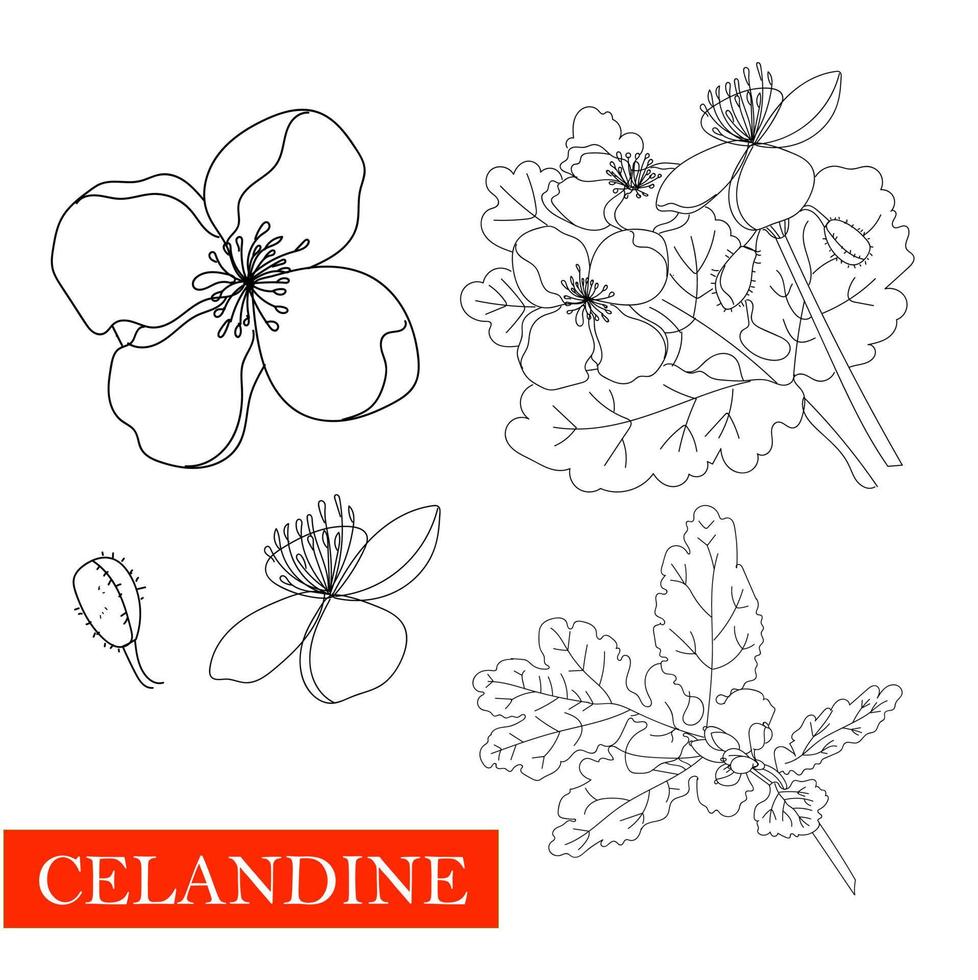The image showcases minimalistic black-and-white pen sketches of various flowers and plants, emphasizing different stages and perspectives. On the left side, there are detailed sketches of flower petals, capturing different views including an unbloomed bud, a side view of a bloomed flower, and a face-on view of the same. Adjacent to these, on the right, is a comprehensive illustration of the entire plant, featuring stems, leaves, and unbloomed buds, depicted as they would naturally appear. Below this, another similar sketch can be found, continuing the detailed botanical theme. In the bottom left corner, a small red rectangle features the word “Celandine” in white uppercase letters, identifying the plant. The entire artwork maintains a monochromatic palette, suggesting a potential use as a coloring page for further detail enhancement.